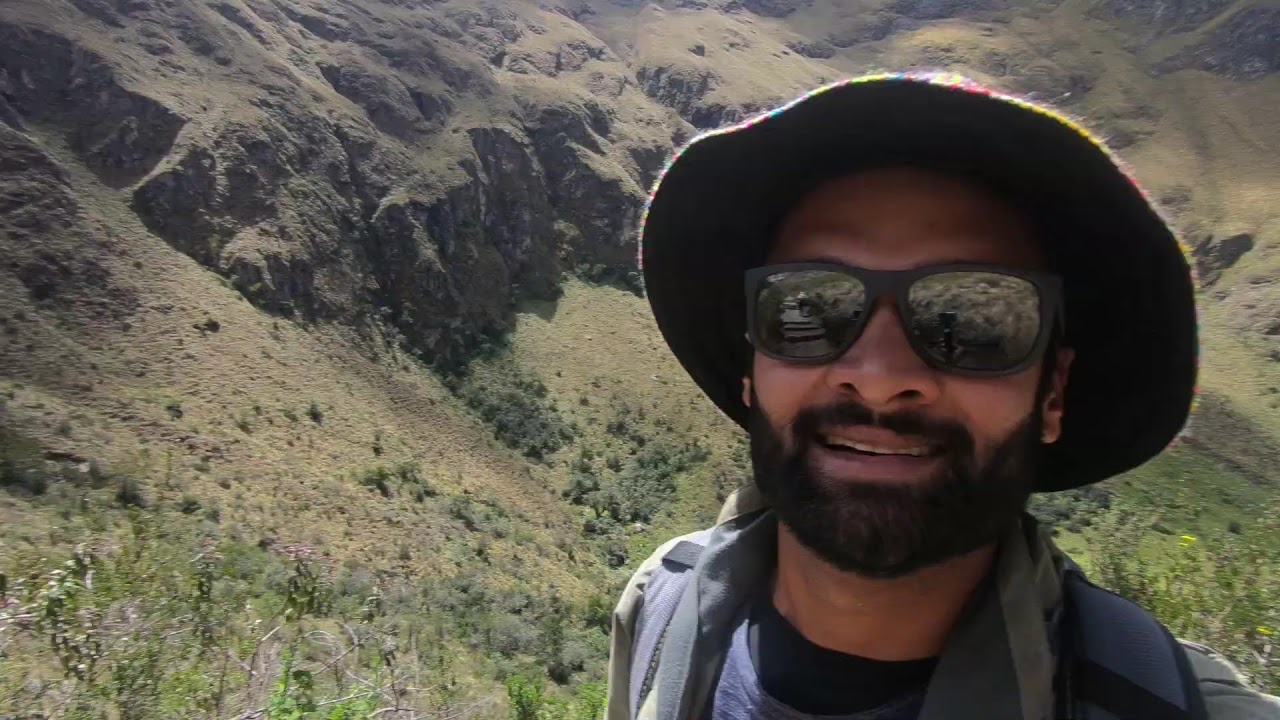In this close-up selfie, a man in his mid-thirties, sporting a well-trimmed thick black beard and mustache, is smiling warmly into the camera. He wears square mirrored sunglasses and a multi-colored sun hat with a round brim featuring shades of yellow, red, and blue. His attire includes a tan windbreaker with a gray collar over a blue t-shirt with a black neckline. A blue-strapped backpack is visible, hinting at his hiking endeavor in this picturesque setting. The backdrop reveals a striking landscape: a mix of green terrain with bushes, small white flowers, and rugged rock formations, indicating he is on or near a rocky hill or mountain. The camera angle suggests he is at a high altitude, offering a glimpse of the valley below, enhancing the scenic nature of this moment.